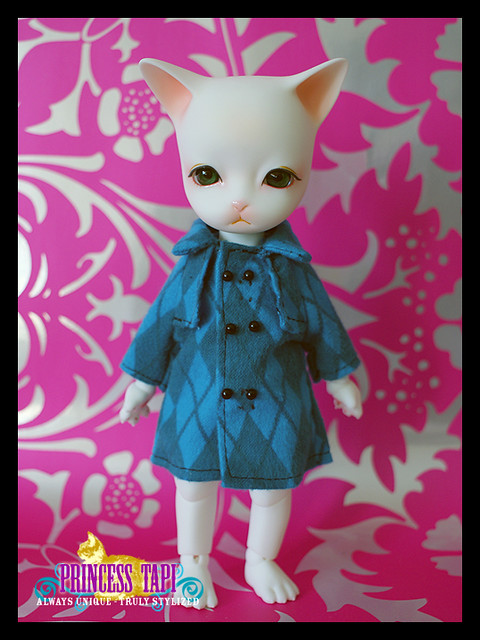The image features a semi-realistic, white plastic cat figurine with a slight pink tint, standing upright on human-like legs. The figure is dressed in a blue trench coat with an argyle pattern in light and dark blue, buttoned up with black buttons. The cat's ears are perked up with pink interiors and it has dark eyes, giving it a lifelike appearance. Its legs are jointed, suggesting some range of motion, which is typical in action figures. The background of the image is pink with a white floral pattern, framed by a solid black border. In the lower left corner, there's a logo that reads "Princess Tappy, always unique, truly stylized," accompanied by a clip art image of an orange cat. The overall setting gives the impression of a product display, possibly for an online advertisement or toy store catalog.